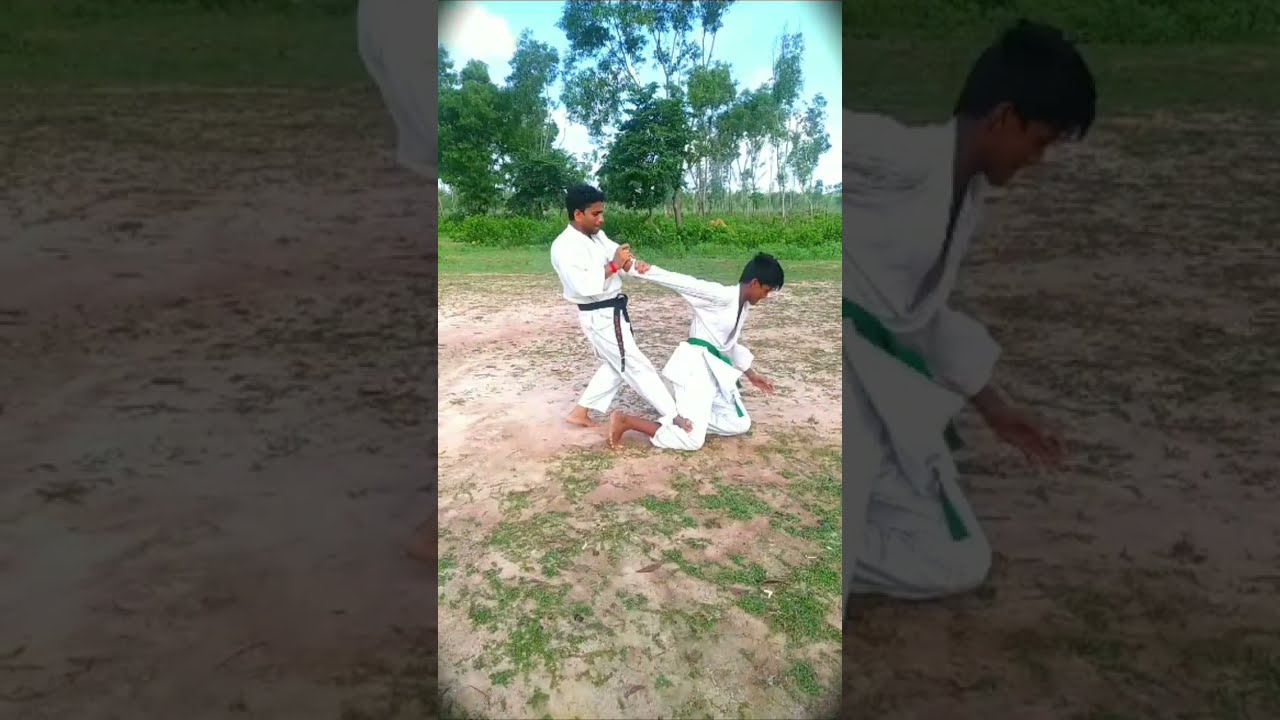The image is a horizontally aligned rectangular picture with a central vertical rectangle depicting two young men engaging in a martial arts practice, likely karate, in an outdoor setting. The young man in the back, dressed in a white uniform with a black belt, is standing and pulling back the right arm of the young man in front of him who is kneeling on the ground, also in a white uniform but with a green belt. The one in back has placed his right leg against the back knee of the kneeling individual, seemingly preparing to take him down. Both individuals appear to be of possibly Indian descent, practicing on a dirt and grassy area with a backdrop of green trees and a blue sky adorned with white clouds. The left side of the image shows a close-up of the standing man’s arm and the dirt ground, while the right side displays a close-up of the kneeling man. These side close-ups are darker and have a faded appearance, blending into the background.